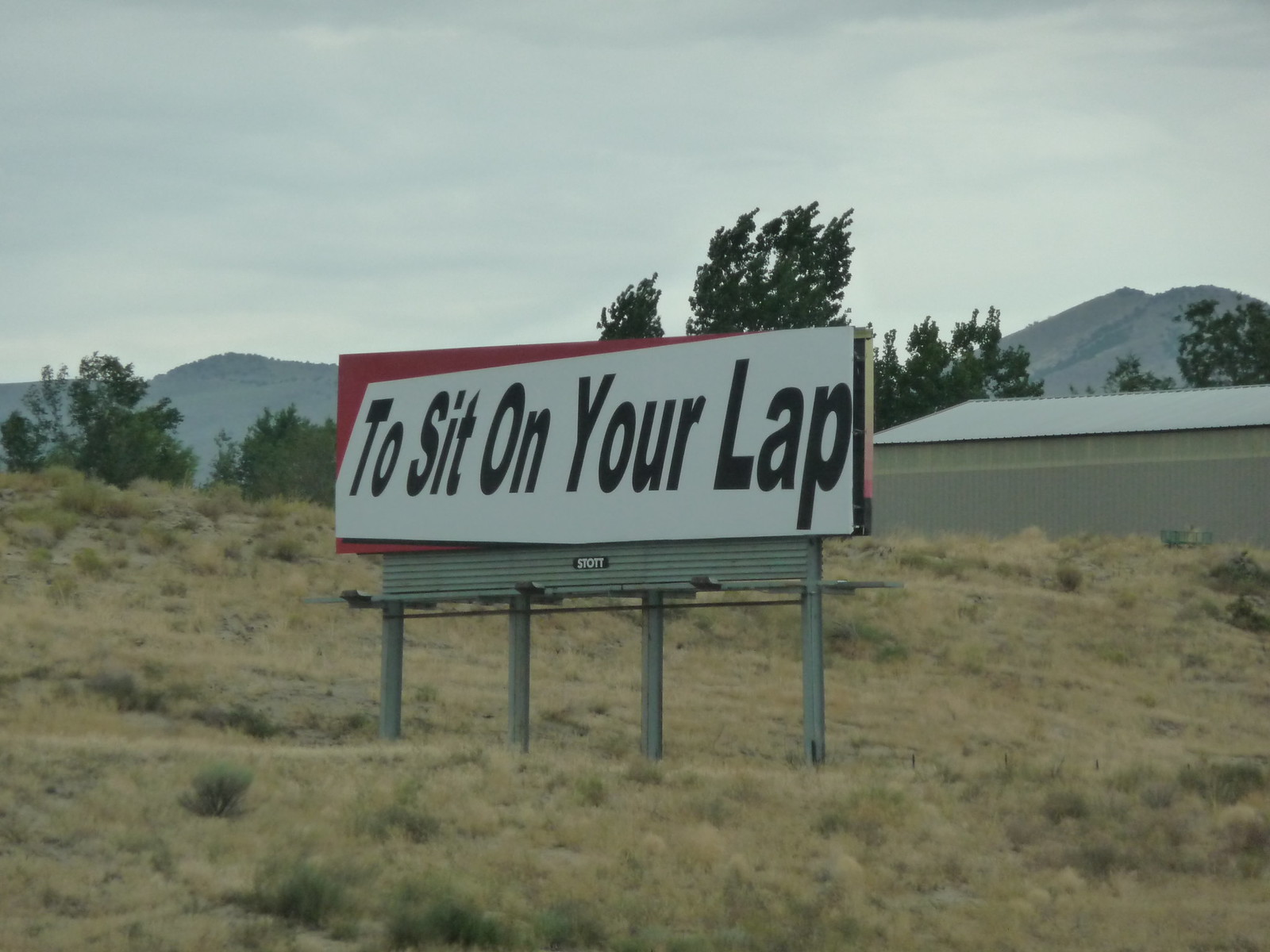In this photograph, we see a billboard situated on a hill covered in dead brown grass intermixed with patches of living green plants and sagebrush. The scene appears to be in a dry, desert-like climate, with a horizon dotted with bushes and a few green trees. Behind the hill, there are dark gray mountains and hills under an overcast, cloudy sky, giving the whole image a very gray and somewhat bleak appearance. The central focus is a small billboard supported by four posts. The billboard features a white rectangle with angled text in black that reads, "To sit on your lap." This white rectangle covers most of a red background behind it. Slightly up the rise, there is a cinder block wall, behind which a tan metal building with a corrugated white roof is partially visible. The background features additional trees scattered around the landscape, completing the rugged and somewhat desolate scene.